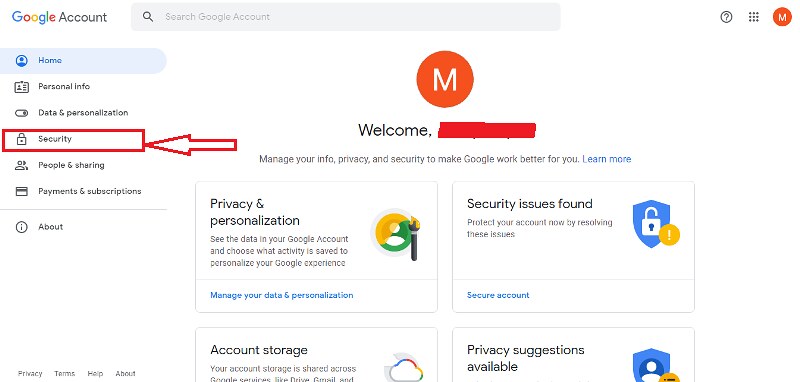The image depicts the Google Account settings page, featuring a comprehensive layout of various options and tools to manage a Google account. 

At the top left, the Google logo is displayed with the letters in the familiar blue, red, yellow, and green colors. Adjacent to the logo is a search bar that includes a magnifying glass icon and the text "Search Google Account" within a grey rectangle.

Across the top right, there are icons for a question mark (help), three vertical dots (more options), and a large red circle indicating notifications.

The left-hand side of the page lists main menu items: "Home," "Personal info," "Data & personalization," "Security," "People & sharing," and "Payments & subscriptions." Below the menu, there is an "About" section marked with an information icon, and a "Privacy & Terms" link.

Underneath the main header, a large red circle highlights the welcome message which reads, "Welcome, [username]." The subheading states, "Manage your info, privacy, and security to make Google work better for you."

The first prominent section on the left is labeled "Privacy & personalization," encouraging users to review their data within their Google Account and choose what activity is saved to personalize their Google experience. This section features a green circle with yellow accents and an icon resembling a person inside a circle, symbolizing user data.

Below this, the "Manage your data & personalization" link is present.

In the upper right quadrant, there is a "Security issues found" alert. This section advises users to protect their account by resolving any identified security issues and features a blue shield with a white lock icon, as well as a yellow circle with an exclamation point for attention.

Lower on the left, the "Account storage" section informs users about their storage usage across various Google services like Gmail. This section displays a cloud icon with a rainbow outline and a statement about shared storage.

Adjacent to this, the "Privacy suggestions available" section is highlighted with a blue shield icon that contains a user avatar, offering tips to enhance account privacy.

Overall, this image provides a detailed and organized representation of the Google Account settings, guiding users through various account management and personalization options.